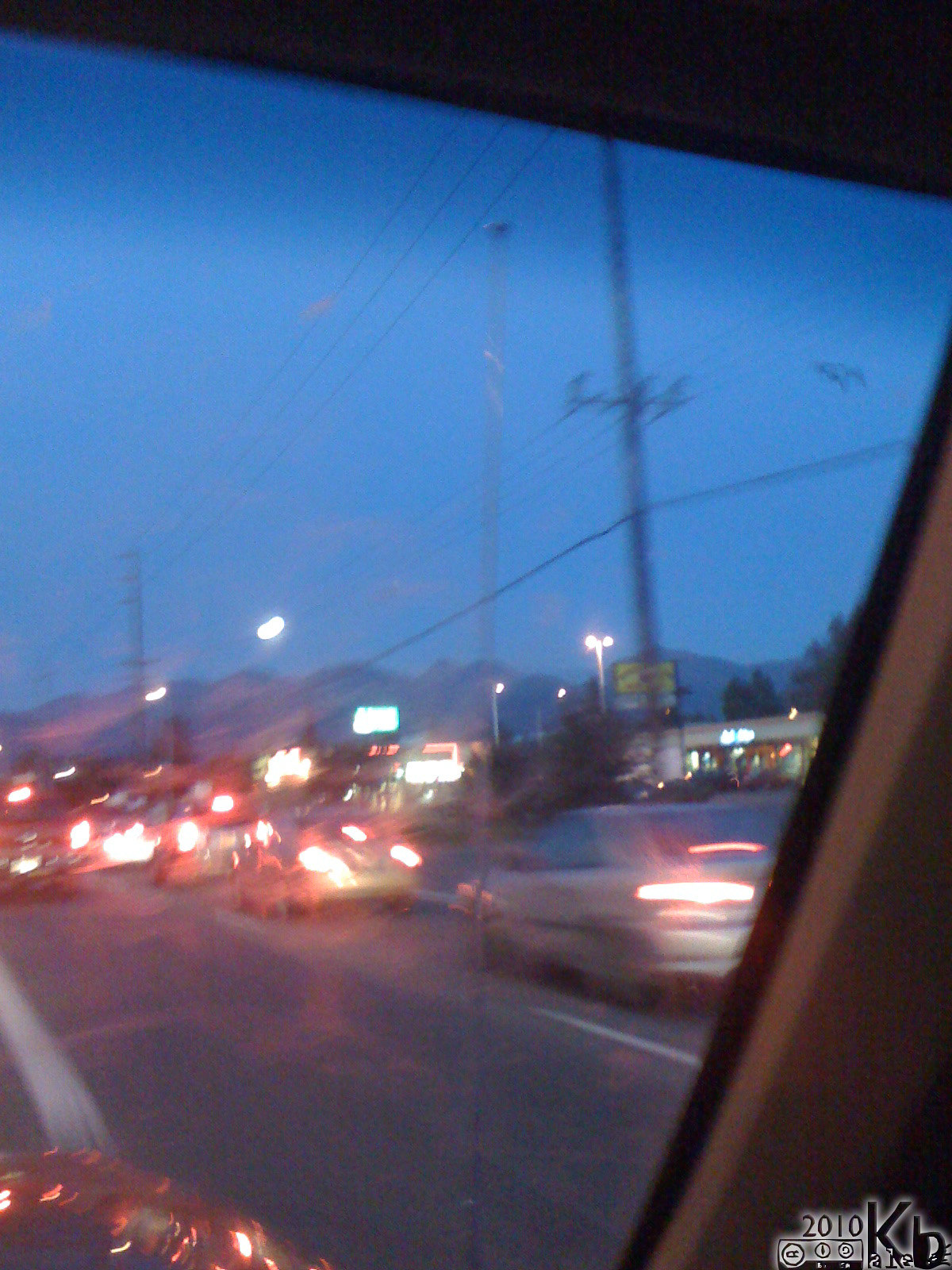The photograph captures an inside view of a car taken during either sunset or sunrise, as indicated by the dark blue sky. In the bottom right corner, a black and white watermark with the text "2010," the letter "K," and various other design elements is visible. The car's tan interior parts, including a pillar and part of the roof, frame the image. Through the window, a dark gray road with white paint lines stretches ahead, populated by numerous blurry cars, likely due to the car's motion or camera shake. These cars, each illuminated with glowing red lights, all appear from the back. Distant mountains create a scenic backdrop, while large power lines and strip malls adorned with illuminated signs add to the urban landscape.